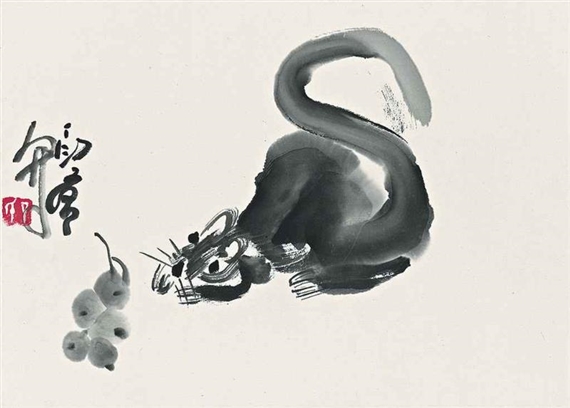The image depicts a detailed and abstract black watercolor painting of a crouching animal, likely a cat, characterized by prominent whiskers, pointed ears, and a long, S-shaped tail curled above its back. The animal, with intense, dark eyes, appears to be inspecting or stalking a cluster of round objects that resemble grapes or nuts on the lower left side of the canvas. The artwork is predominantly black, gray, and white, with a starkly contrasting pop of red text in what seems to be Japanese or Chinese characters on the left side, contributing to its Asian aesthetic. The scene is set against a pristine white background, and the artist's signature is visible alongside the red stamp, adding a unique and cultural touch to the composition.